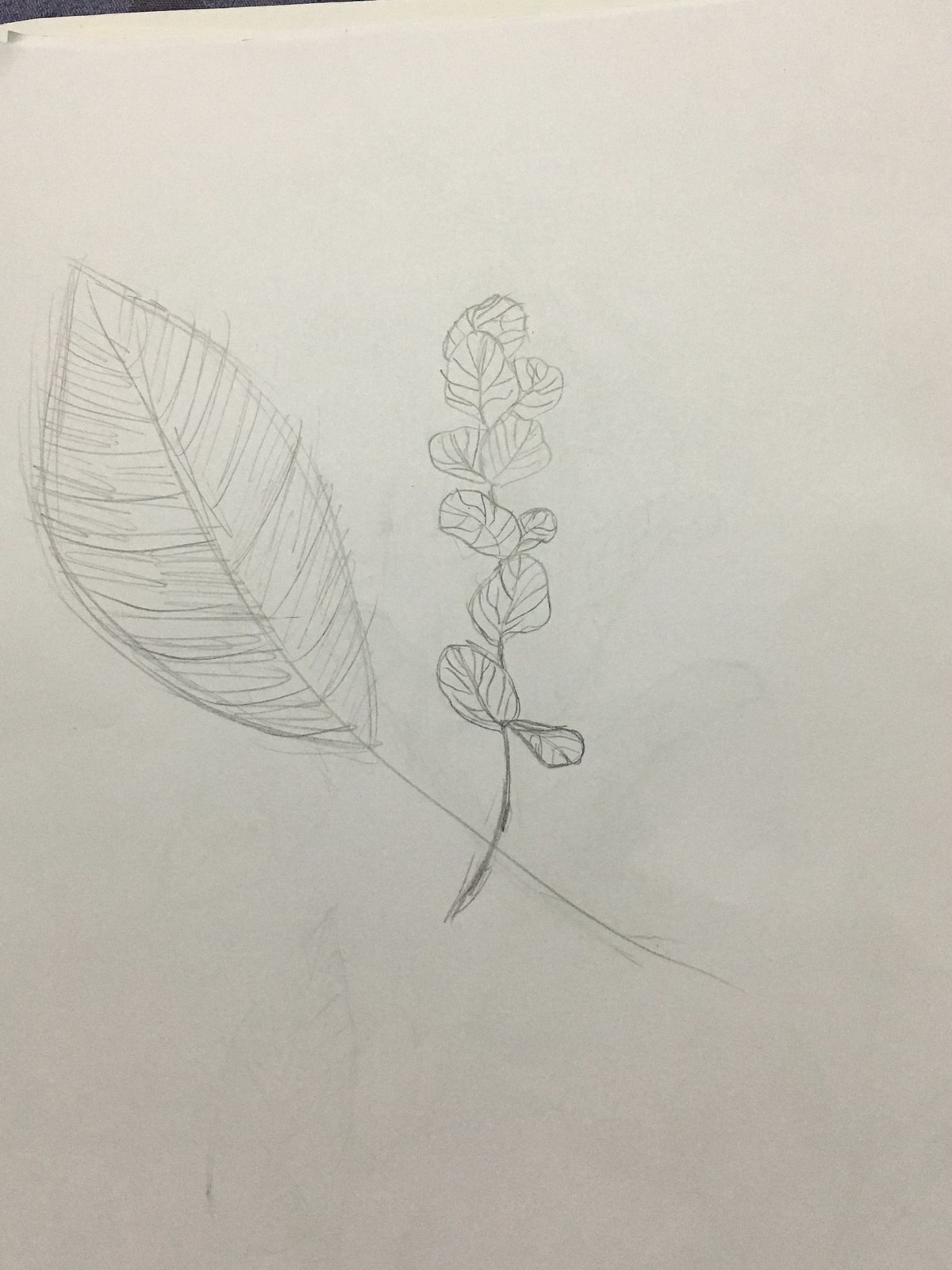This detailed pencil sketch on white paper features a large, prominent leaf and a smaller branch of leaves, crafted with careful attention to detail. The single, oblong leaf, pointy at both its top and bottom, occupies the left side of the composition and is angled upward towards the left corner. Its thin stem crosses at the bottom with the stem of the smaller branch, which extends upward towards the top of the page. This branch showcases around ten smaller, circular leaves, each with delicate lines indicating veins. The sketch varies in pencil shading, with the smaller branching leaves appearing slightly darker, adding depth and contrast to the overall image.